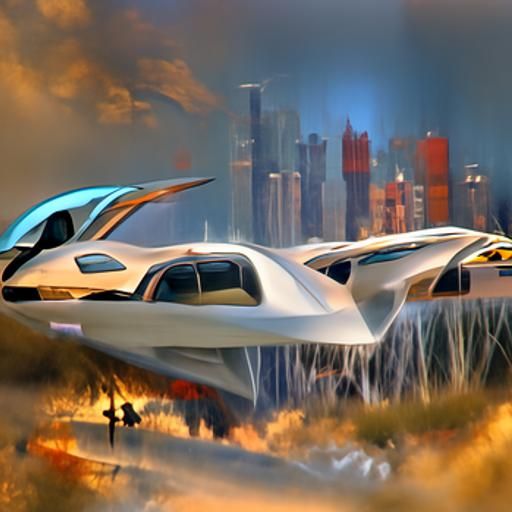This image features a computer-generated, futuristic airship dominating the central portion of the frame. The airship is predominantly a shiny silver and whitish-gray color, with sleek black windows peppered across its surface. On its top, there's a distinctly blue-outlined, raised cockpit area and downwards, a triangular-shaped fin exhibits a recessed section. The scene below the airship is dramatic, with the ground appearing to be engulfed in intense flames, surrounded by burning trees with white trunks and billowing black smoke. In the background, a city skyline emerges through a haze; the buildings, varying in color from blue and red to gray and orange, stand tall. Some have sharp, pointed tops while others are flat, and they too are partly obscured by the pervasive smoke. The sky above transitions from blue to gray, intensifying the chaotic atmosphere with vibrant orange and black clouds, echoing the turmoil below.